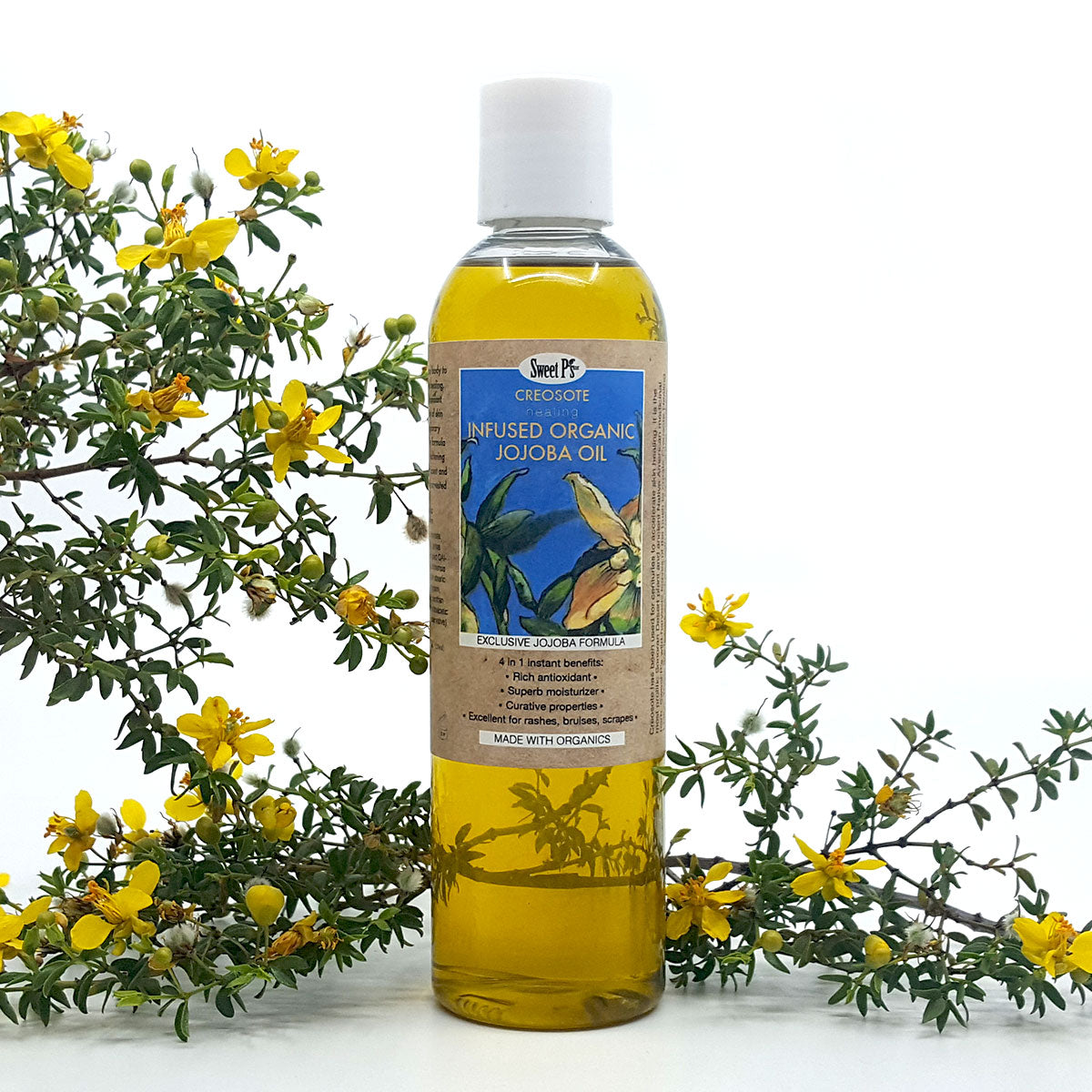The image features a transparent bottle filled to the brim with golden organic jojoba oil. Topped with a white cap, the bottle displays a tan label that prominently features a blue illustration of the jojoba plant, with green leaves and yellow flowers. The label reads "Sweet Peas Infused Organic Jojoba Oil" in vibrant yellow letters. Below, it is noted that the product is "Made with Organics." Behind the bottle, more jojoba plants with petite yellow flowers and green foliage can be seen blending with the white surface and background. The product is marketed as having "Four-in-One Instant Benefits," including rich antioxidants, superb moisturizing properties, creative properties, and excellent efficacy for treating rashes, bruises, and scrapes.